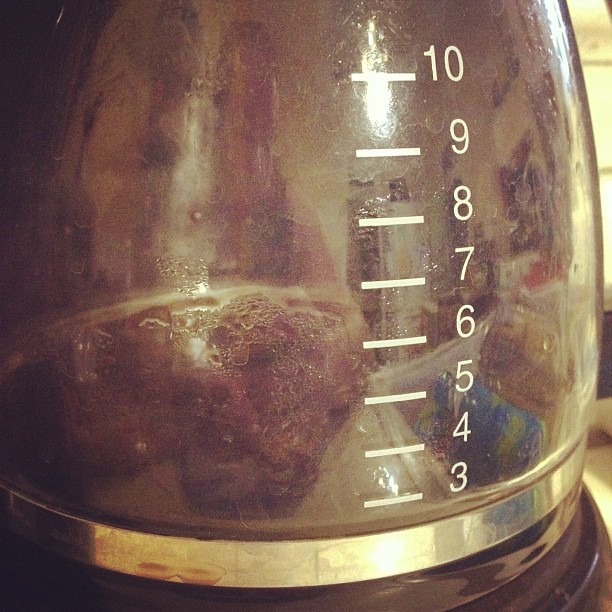This square image is a poorly taken, slightly blurry color snapshot of the carafe, or glass coffee pot, part of a coffee maker, bathed in tungsten lighting. The shot zooms in on the glass portion, featuring white horizontal lines with numbers from 3 to 10 to the right, indicating the number of cups of coffee that can be made. The pot's base is a silver or gold-colored metal with a black bottom, which reflects its surroundings. The glass is somewhat clear but has moisture inside, possibly indicating an old or unclean state, with some texture suggesting water at the bottom. The predominant colors in the image are light brown, bright yellow, black, and light gray.